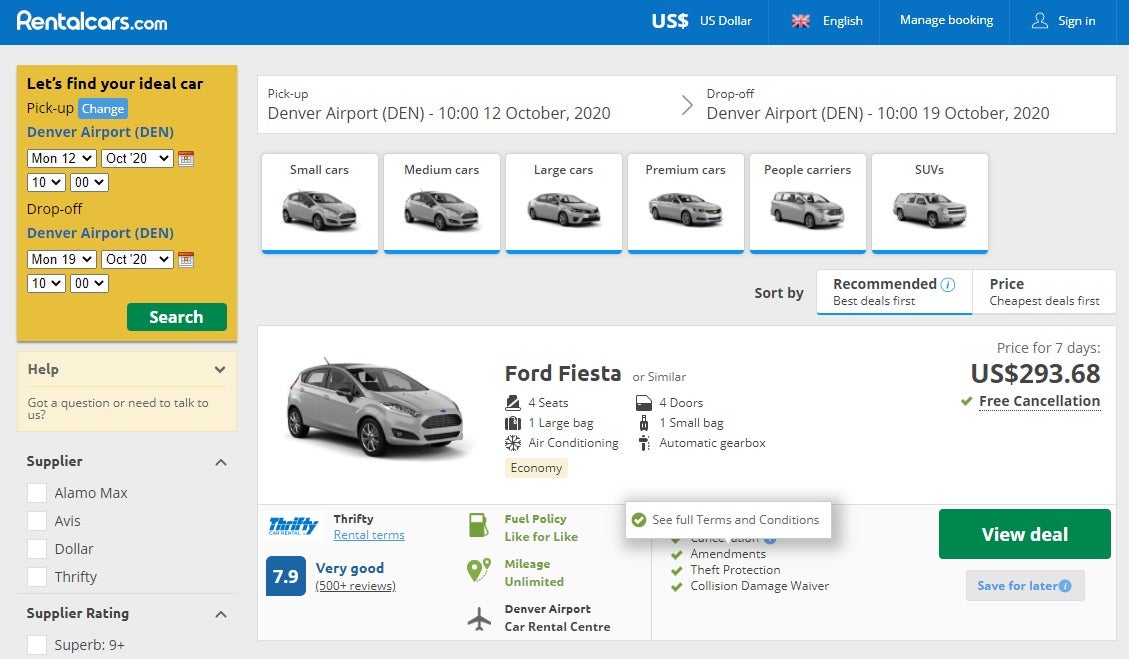"On the rentalcars.com homepage, there is a banner that reads 'Let's find your ideal car.' The search module is set with 'Pick-Up Location' as Denver Airport (DEN) and the 'Date and Time' fields filled out. The pick-up date is scheduled for Monday, 12th October 2020 at 10:00 AM, and the drop-off is set for Monday, 19th October 2020 at 6:03 PM. To the right, a 'Search' button awaits action. Below, different car categories are displayed: Small Cars, Medium Cars, Large Cars, Premium Cars, People Carriers, and SUVs. For instance, a Ford Fiesta is listed with the rental period from 12th to 19th October 2020, detailed with a price of $293.68. At the bottom right corner, a 'Help' button is visible for further assistance."